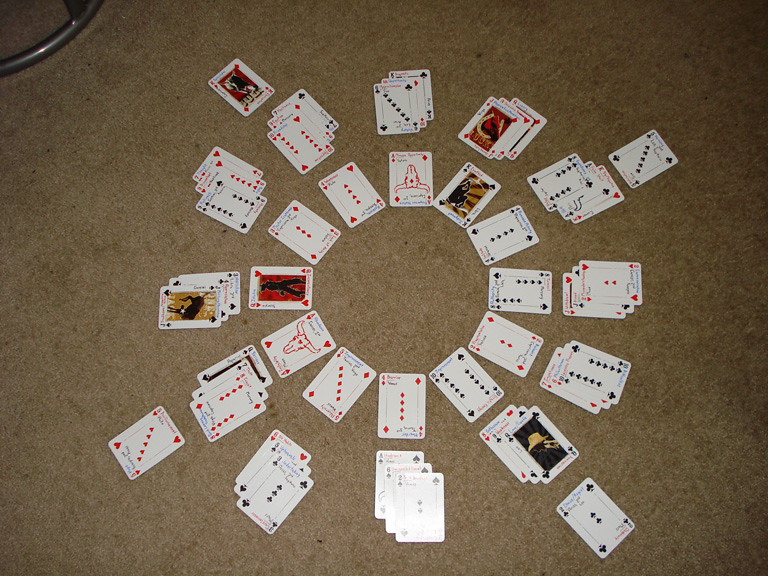On a brownish floor, possibly wood or a carpet, lies an intricate arrangement of playing cards. Near the top left corner is a round, metallic base, possibly the pedestal of a bar stool. In the center of the display are 12 playing cards meticulously arranged in a tight circle. Surrounding this inner circle is a larger circle comprised of 12 or 13 stacks, each consisting of three cards. Four single cards are placed outside of these circles, each occupying a corner position in the layout—upper left, upper right, bottom left, and bottom right. The cards appear to be part of a standard deck featuring hearts, diamonds, and spades. Some cards depict images of a bull with horns, and specific cards are identifiable, including a three, a two, and a jack of hearts. The arrangement seems to be an artistic display meant to showcase the entire deck of 52 cards.